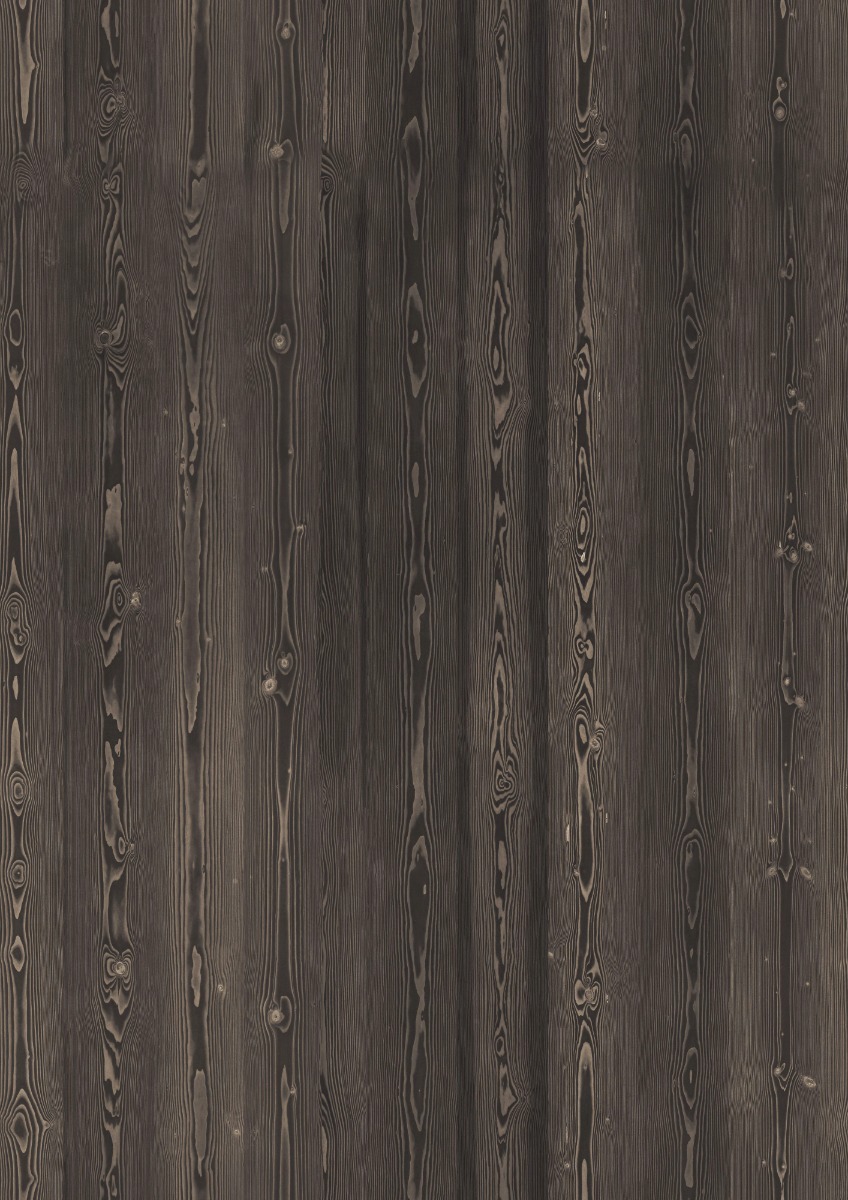The image depicts a very simplistic yet detailed photo of a piece of wood paneling, filling the entire frame and offering no context for its location. The wood features very pronounced vertical grains, varying in width from several inches to six or eight inches. The color is a dark, weathered gray, almost verging on black, with lighter, whitish accents highlighting the wood's intricate veins and knotted pieces. The grain patterns appear almost artistic, resembling slender, tribal symbols or flowers, as if specifically enhanced with paint. The overall appearance is of a deeply textured, weathered wood that evokes both natural resilience and artistic enhancement.